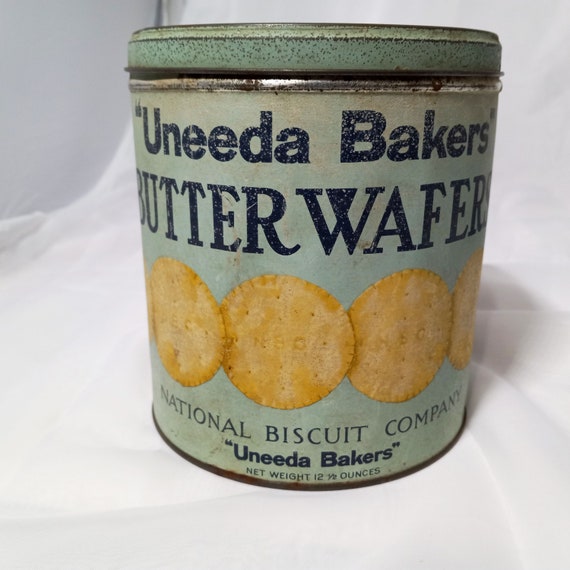This antique metal tin can, with its lid still intact, appears to have been carefully staged for display, likely for sale or advertisement purposes. The can is an aged, somewhat faded teal color, featuring noticeable wear such as scuff marks, rust, and patches where the paint has worn off. The front prominently displays "UNEDA BAKERS" in quotes, followed by "BUTTER WAFERS" in all capital letters, and "NATIONAL BISCUIT COMPANY" at the bottom. The can showcases images of the buttery wafers or crackers, which are round in shape. The net weight is marked as 12.5 ounces. This vintage item, perhaps never opened, rests on a white draped fabric, adding to its nostalgic charm.